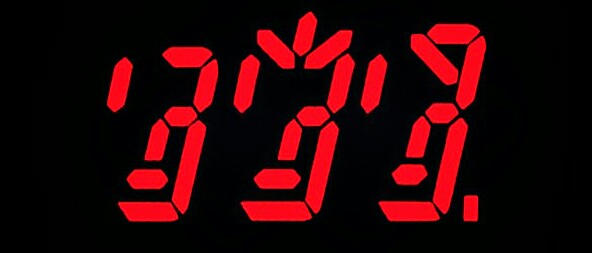This image depicts the face of a digital clock with an unusual and garbled display. Instead of the typical format showing hours and minutes separated by a colon (e.g., "13:33"), the numbers appear jumbled and resemble nonsensical symbols. The characters are an array of irregular red shapes, suggesting that the digital figures have been either manipulated or distorted. The far-left digit appears as though it might have originally been a "1", followed by three figures that resemble "3"s. However, each of these digits has been altered, contributing to the overall impression of randomness and disarray. The effect transforms what would ordinarily be a clear time display into a chaotic arrangement of shapes.